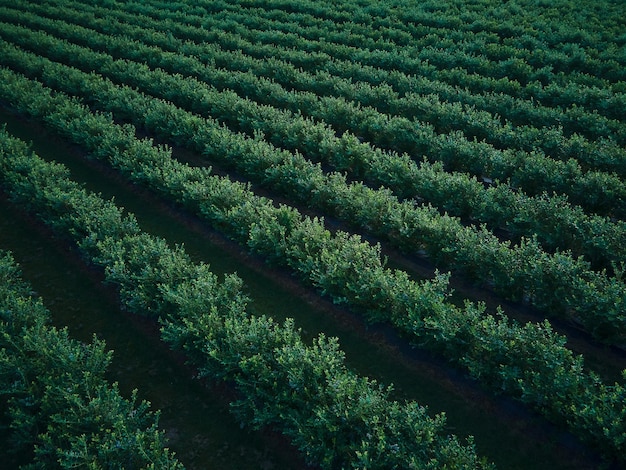The image presents a well-maintained grid of greenery, consisting of 13 to 20 rows of bushes that appear tall and well-hedged. Captured from a height of about 20 feet at a slight angle, the photograph highlights a realistic outdoor setting, presumably during the day, as suggested by the good lighting. Each row of lush, deep green bushes is interspersed with darker shaded walkways, possibly grass or dirt paths, which may be lined to prevent weed growth. The uniform and meticulously trimmed appearance of the plants, possibly vegetables like potatoes, suggests they are cultivated, giving the impression of a farm or garden. The image exclusively showcases these rows of greenery, devoid of any other objects or text, creating a simple yet striking aerial view of agricultural precision.